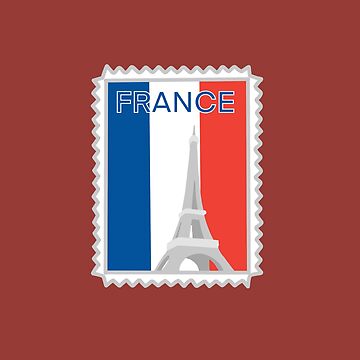The image displays a rectangular postage stamp placed against a dark maroon background. The stamp's edges are ridged, with a distinctive white frilly pattern surrounded by a light gray outline that defines its shape. Within the stamp, the flag of France is prominently featured, slightly elongated to cover the entire central area. The flag is composed of three vertical stripes: blue on the left, white in the center, and red on the right. At the top of the stamp, the word "France" is written in bold blue letters with a white outline.

Dominating the middle to the upper section of the stamp is a simplified, cartoonish rendering of the Eiffel Tower. The tower transcends the boundary between the white and red stripes, with its base starting near the bottom center of the stamp and its tip extending upwards, nearly reaching the letter "C" in "France." The Eiffel Tower is depicted in medium and light gray colors, adding a three-dimensional effect to the image.